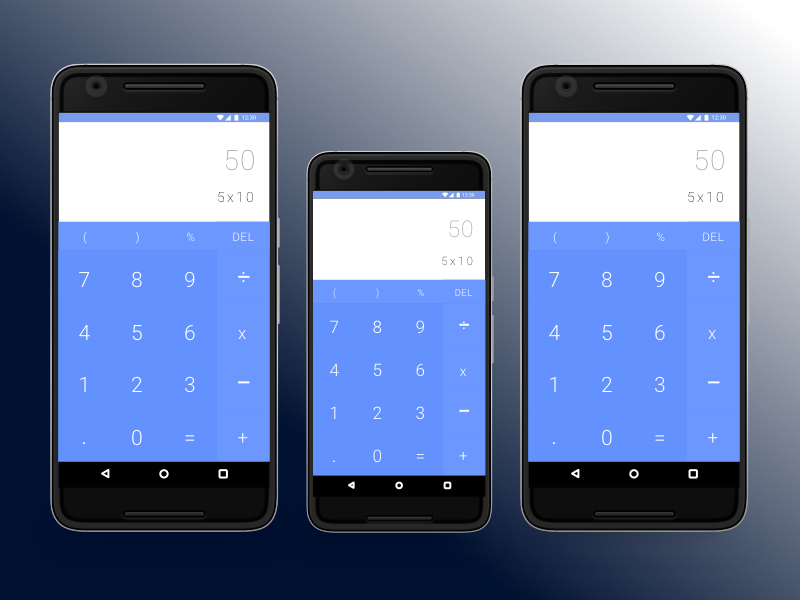The digital collage features a gradient background that transitions from a white corner in the top right, through shades of gray, and culminates in a dark navy blue in the bottom left. At the center of this backdrop are three iPhone screens, each displaying identical calculator interfaces. The iPhones differ slightly in size; the two on the left are marginally taller and wider than the one in the middle. Each screen shows a thin blue line at the top adorned with white icons in the right corner. Below this line lies a wide white rectangle that reads "50" to the right, with "5 times 10" in gray. The calculator interface comprises buttons in various shades of blue, featuring the numbers 0 through 9 alongside mathematical operators like division, multiplication, subtraction, and addition. The collective appearance of the number keys and background elements display hues ranging from light blue to a deeper, almost purple blue. The gradient background and the vivid blue calculator displays create a visually cohesive and striking image.